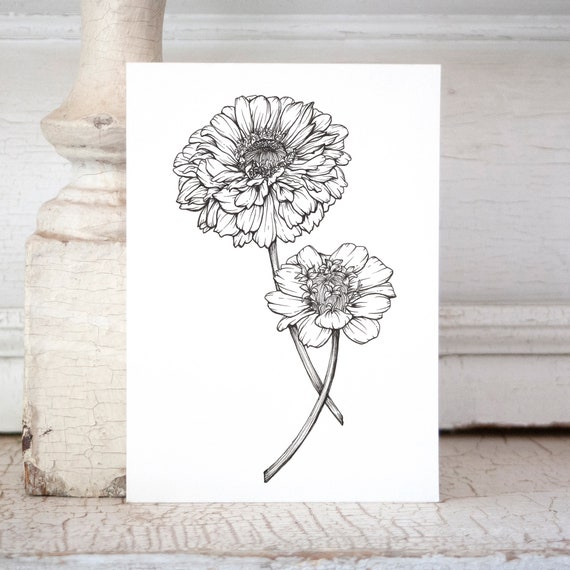This detailed image shows a simple yet intricate pen and ink drawing on a white piece of paper, featuring two chrysanthemums, or possibly daisies, in black and white. The larger flower is fully bloomed and positioned at the top left, while the smaller flower, with some buds emerging, is slightly below and to the right. The stems of the flowers elegantly cross each other. This drawing is set against a background of aged, cracked, white-painted wood, which could be part of a shelf, mantel, or possibly an old banister or spindle. The wood’s worn, antique appearance adds a nostalgic and rustic charm to the scene. The overall composition blends the delicate artistry of the flowers with the textured, vintage character of the wooden background, creating a striking and harmonious visual.